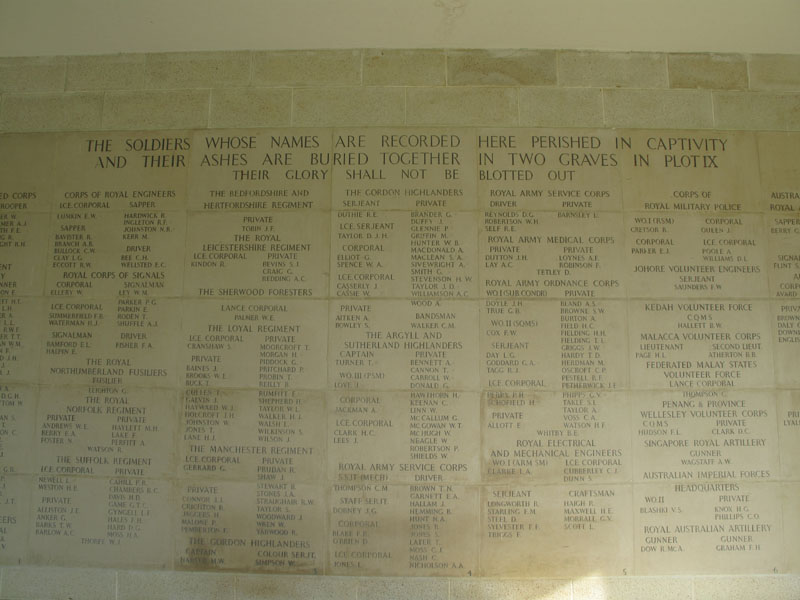This photograph captures a detailed and somber war memorial, featuring a brick wall adorned with tan or cream plaques, slightly shadowed by natural light. The top of the plaques bears a poignant inscription in black, capital letters: "THE SOLDIERS WHOSE NAMES ARE RECORDED HERE PERISHED IN CAPTIVITY AND THEIR ASHES ARE BURIED TOGETHER IN TWO GRAVES IN PLOTIX. THEIR GLORY SHALL NOT BE BLOTTED OUT." Beneath this tribute is a lengthy and meticulously organized list of names of the soldiers. The names are arranged by regiment and corps, including the Royal Regiment, the Argyle and Southern Highlanders, the Royal Army Service Corps, the Corps of Royal Engineers, and the Sherwood Foresters. Each name and rank, such as Private Tobin J.F. from the Royal Leicestershire Regiment, is inscribed in black capital letters, honoring over a hundred individuals who made the ultimate sacrifice. The solemnity and reverence of the memorial are palpable, conveying a powerful tribute to the fallen soldiers.